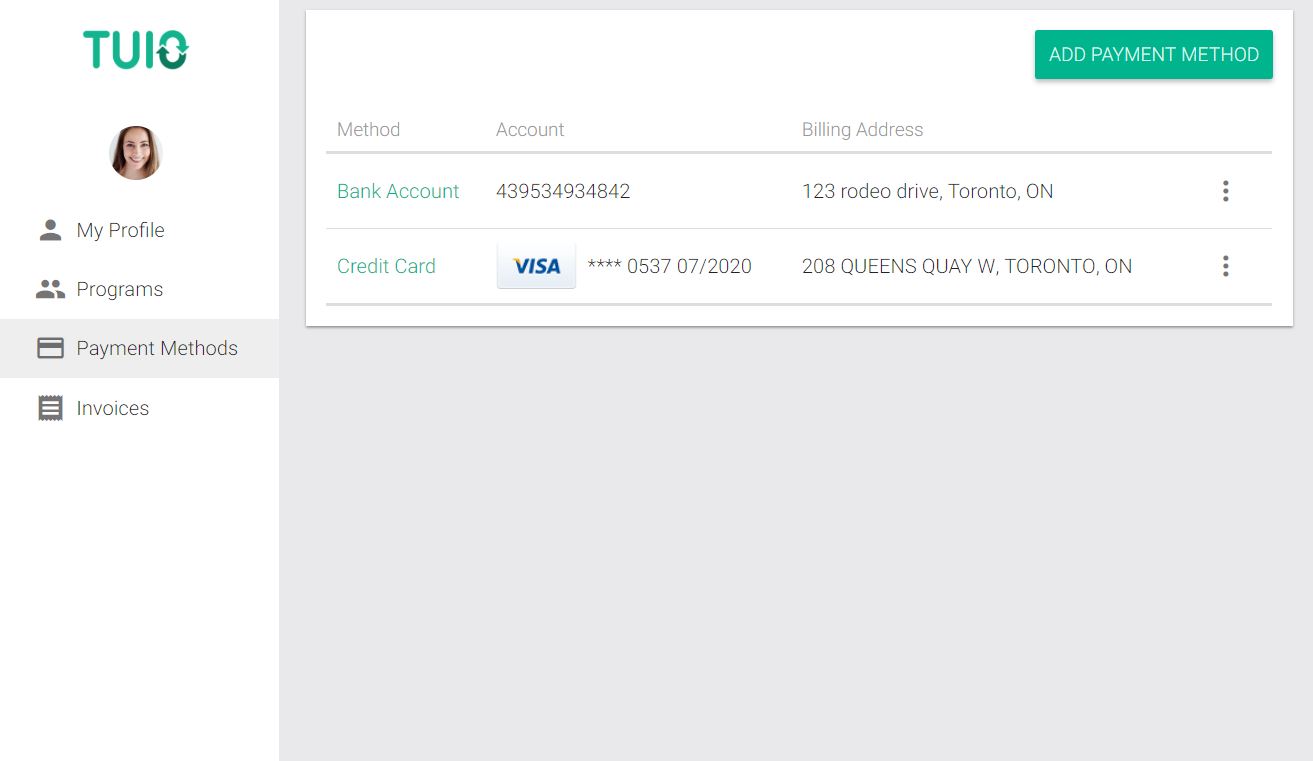The image features a light blue background split into two main sections. On the left side, there is a prominent white box displaying the text "T-U-I-O," where the "O" is stylized with a curved arrow pointing downwards and another curved arrow pointing upwards. Below this, a circular icon contains a profile picture of a lady, leading to options labeled "My Profile," "Programs," "Payment Methods" (highlighted in blue), and "Invoices."

On the right side of the image, set against the same blue background, there is another white box with sections labeled "Method," "Account," and "Billing Address." In the upper right corner of this box, a green button reads "Add Payment Method." The box lists a bank account with partial account information and the address "123 Rodeo Drive, Toronto, Ontario," accompanied by an ellipsis icon. Below, another section identifies a Visa credit card with partial card information and the address "208 Queens Quay W, Toronto, Ontario," also accompanied by an ellipsis icon. A blue line separates these two payment sections within the white box.